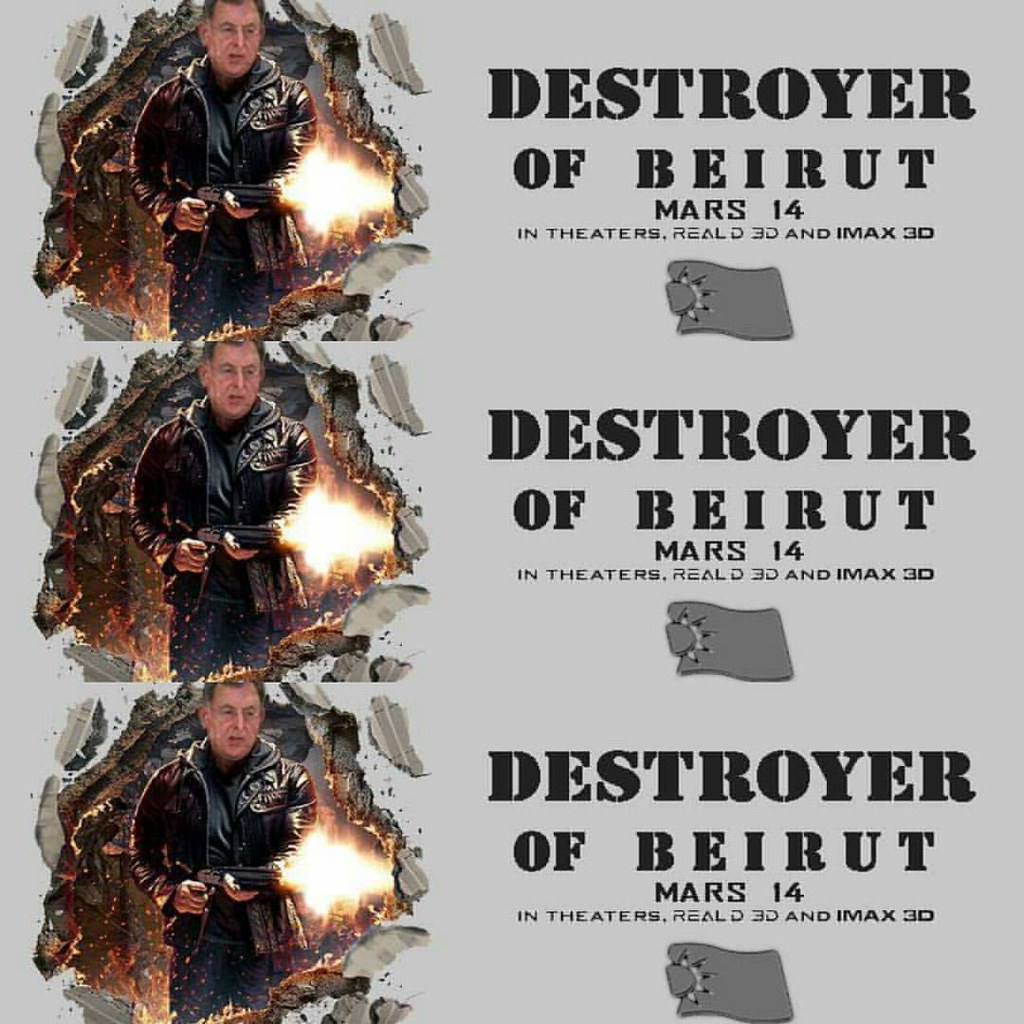The movie poster for "Destroyer of Beirut," set against a grey background, features a dramatic scene of a middle-aged Caucasian man in a red leather jacket and grey hoodie blasting through a wall with a shotgun, debris scattering everywhere. Fiery blast is visible from the shotgun. The right side of the poster prominently displays the title "Destroyer of Beirut," the release date "Mars 14" (March 14th), and mentions that the film will be available in theatres in Real 3D and IMAX 3D. The striking composition is multiplied three times in a merged vertical column, enhancing the impactful visual.